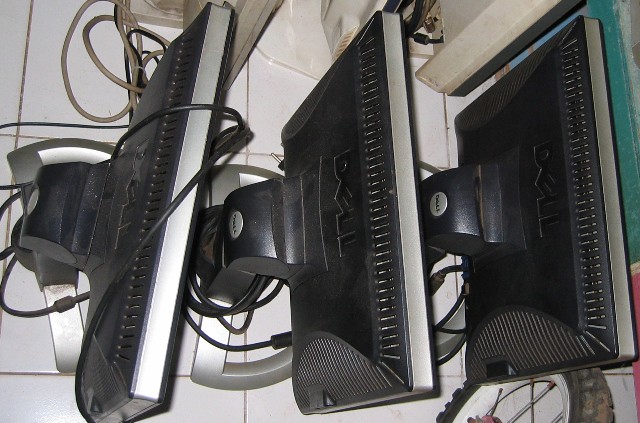This photograph features three Dell computer monitors placed on a white tile floor, possibly in a corner or garage. Each monitor has a black back with "Dell" prominently displayed, a gray border around the screen, and a silver base. Numerous cords, including power and HDMI, are wrapped around the bases and sprawled out to the side. Positioned in a row, the monitors also have black attaching arms holding them. The angle of the shot suggests it was taken from above, looking down towards the monitors. In the bottom right corner of the image, there's a bicycle wheel with dirt marks on it, indicating it might have been recently used. This additional detail, coupled with the scattered electronics, hints that the picture could have been taken in a garage space.